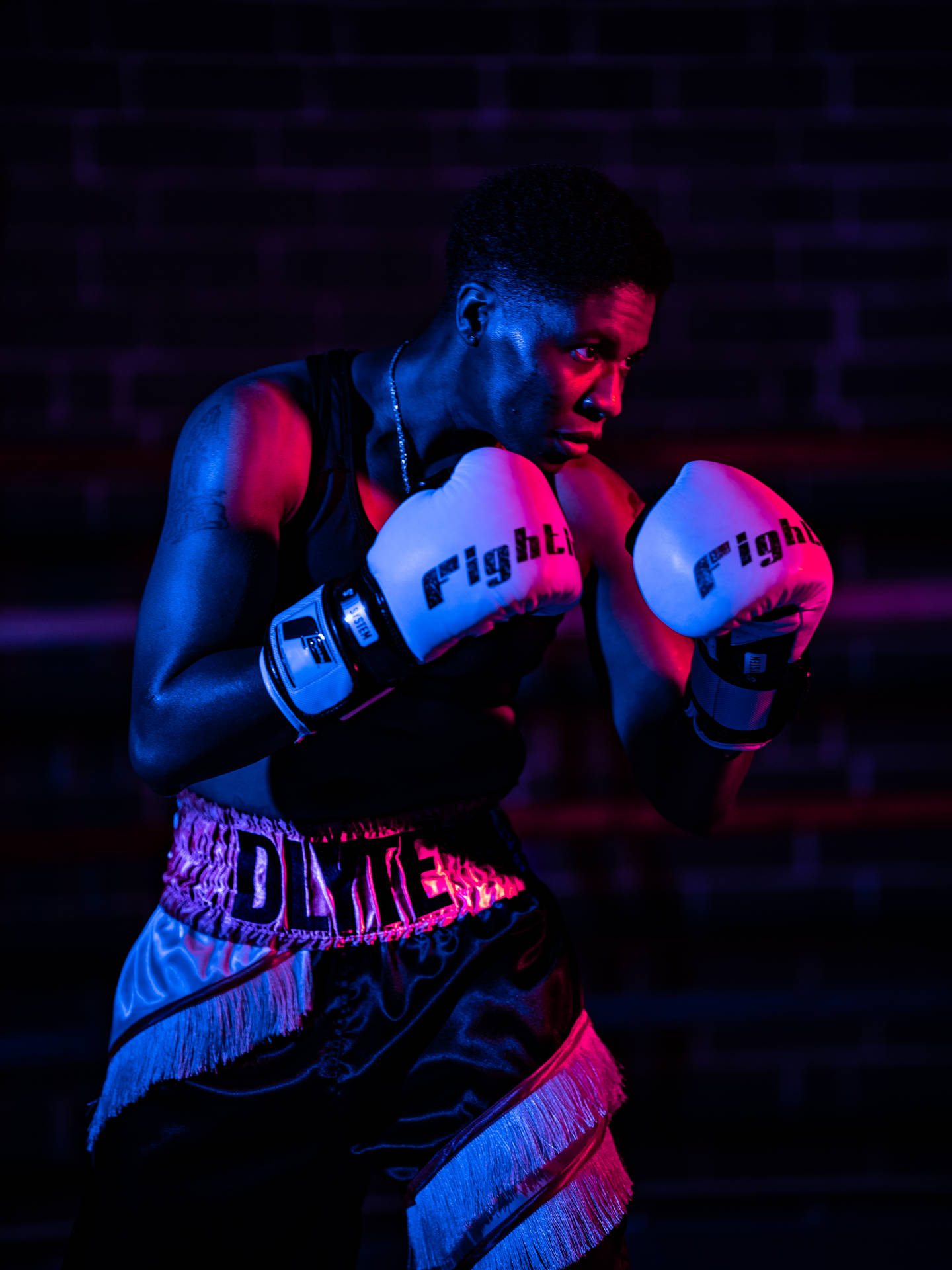The image features a Black boxer standing in a fighting stance with raised fists. The background is dark, creating a stark contrast with the vividly colored lighting that illuminates the boxer, casting a blue hue on the left side and a red tint on the right side of his body. He wears a black tank top and distinctive boxing gear that includes white boxing gloves with black wristbands, bearing the word "Fight" on them. The boxer's shorts are eye-catching, adorned with pink and black stripes and fringes, and feature a pink waistband emblazoned with the letters "D-L-Y-F-E." Completing the look is a gold necklace that glints against the contrasting light. The short tassels line the trunks, adding a dynamic element to his attire, swirling from the front center to the back and around the legs. The image is further punctuated by subtle details like possible ring ropes in the background, enhancing the setting’s ambiance.